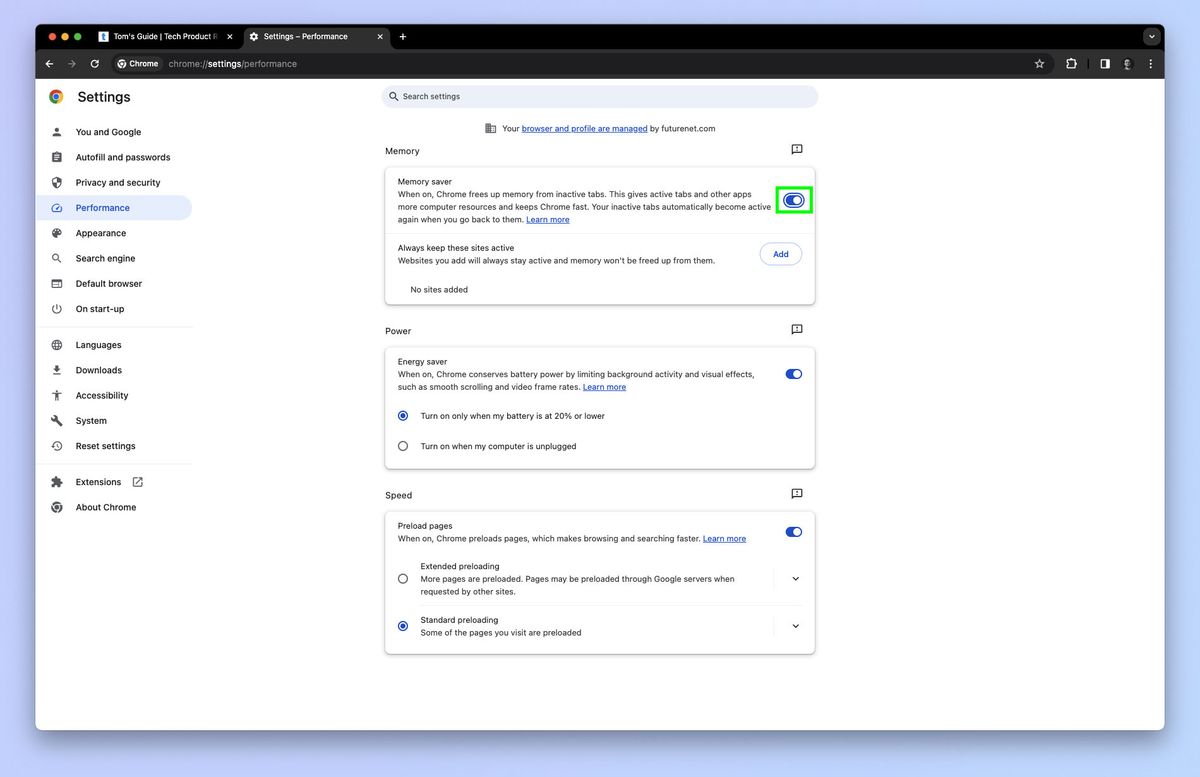This image depicts a detailed view of the settings page within the Google Chrome browser. The content is organized into a left sidebar and a primary content area. In the left sidebar, an array of categorized settings is listed: 

1. "You and Google"
2. "Autofill"
3. "Privacy and Security"
4. "Performance" (this section is currently selected and highlighted in blue)
5. "Appearance"
6. "Search Engine"
7. "Default Browser"
8. "On Startup"
9. "Languages"
10. "Downloads"
11. "Accessibility"
12. "System"
13. "Reset Settings"
14. "Extensions"
15. "About Chrome"

At the top of this sidebar is the main header labeled "Settings."

The main content area on the right side focuses on "Performance Settings." At the top, there is a search bar with the placeholder text "Search settings." Directly below, it notes that "Your browser and profile are managed by FutureNet.com."

The "Performance Settings" section is divided into three parts:

1. **Memory**:
   - "Memory Saver": A description explains that when this feature is enabled, Chrome frees up memory from inactive tabs, giving more resources to active tabs and other applications. Inactive tabs will automatically reactivate when revisited. A toggle switch for "Memory Saver" is on and highlighted in blue, outlined by a green box.
   - "Always keep these sites active": Users can specify websites that should remain active at all times. A button to add sites is present, but currently, no sites are added.

2. **Power**:
   - "Energy Saver": When enabled, this setting conserves battery by limiting background activity and visual effects like smooth scrolling and video frame rate. The toggle switch is enabled and blue, set to activate when the battery is at 20% or lower.

3. **Speed**:
   - "Preload pages": This setting, when enabled, allows Chrome to preload pages to enhance browsing and searching speed. The toggle switch is on, with two preloading options visible—"Extended Preloading" and "Standard Preloading," with the latter selected.

This detailed layout ensures efficient navigation and customization within the Chrome browser, providing users with various tools to enhance performance, conserve battery life, and speed up browsing.